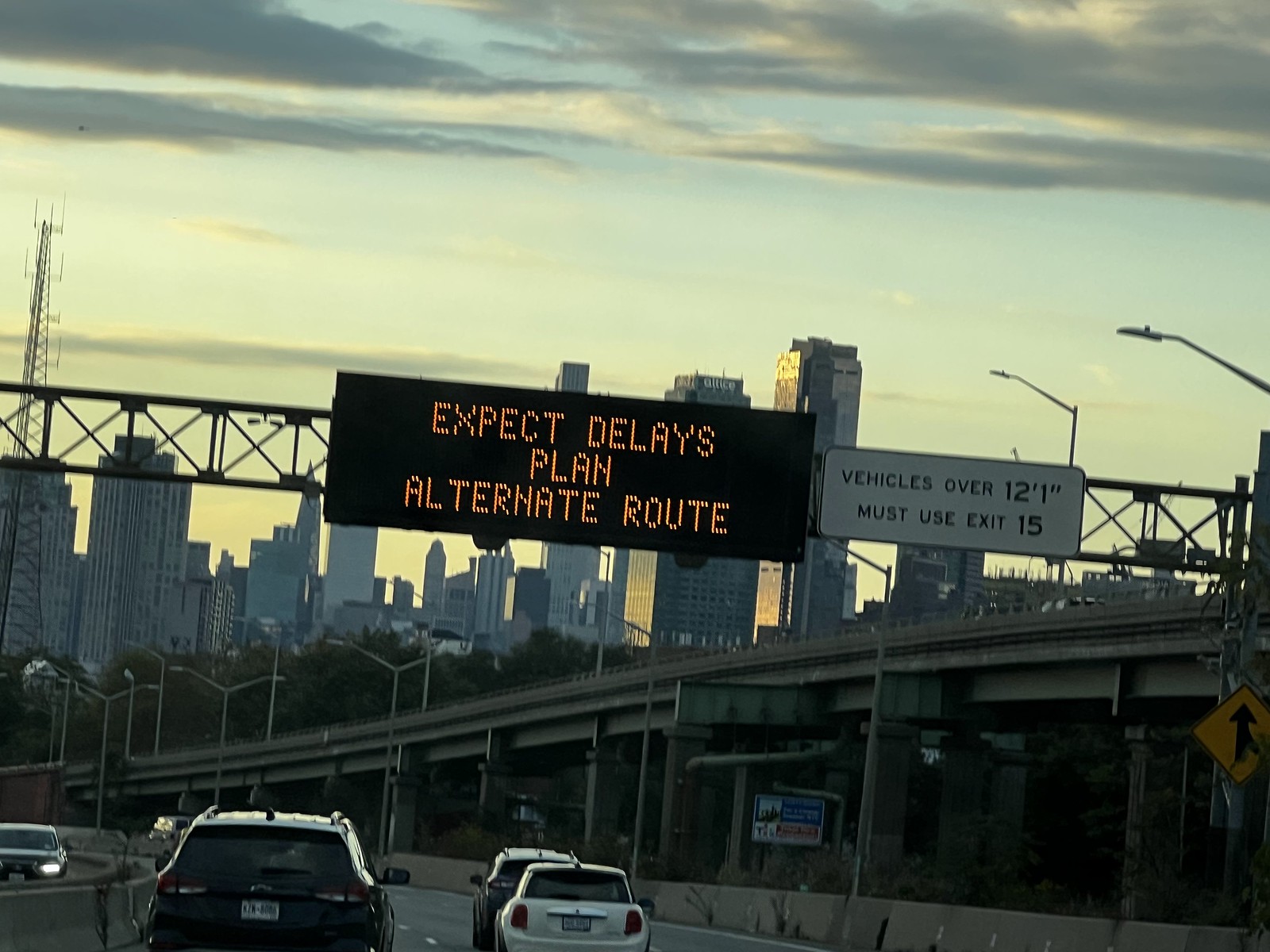The photo captures a scene taken from a car on a major highway in what is evidently a bustling city, as depicted by the towering skyscrapers in the background. A digital sign spanning three lines reads "Expect delays, plan alternate route," while another adjacent sign to the right reads "Vehicles over 12 foot 1 inch must use exit 15." The evening sky, marked by dark clouds, adds a dramatic contrast to the cityscape. On the highway, a black SUV and a white car drive ahead, while an elevated roadway looms above. Additionally, a yellow sign near the base of the pole supporting the other signs features an arrow with a split in it, indicating traffic directions. The barrier separating the highway lanes is visible, with vehicles traveling in the opposite direction also captured in the frame.